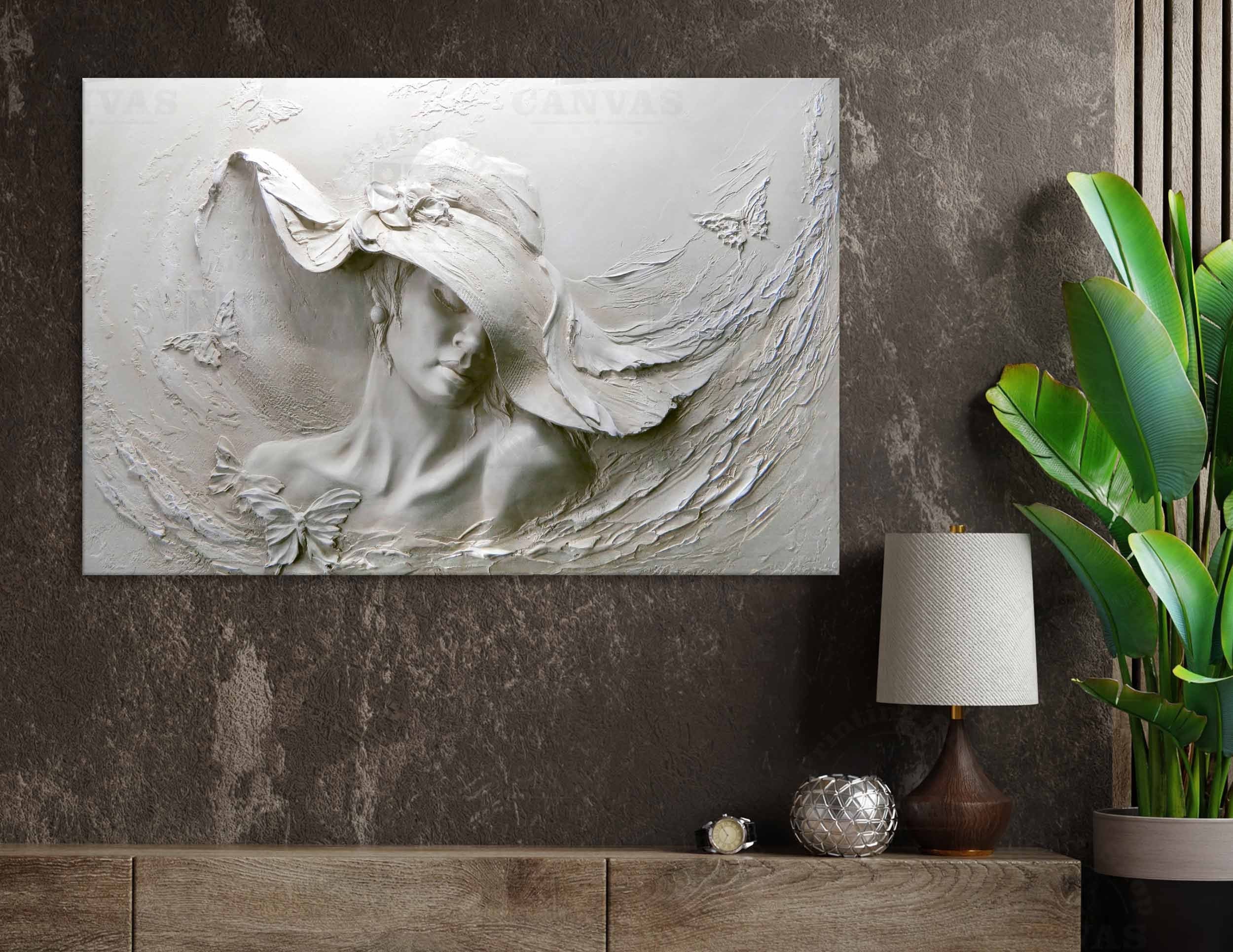The image depicts an elegant interior room with a textured grey wall as the backdrop. Adorning the left side of the wall is a three-dimensional art piece of a woman. The intricately detailed sculpture shows the woman in a large hat adorned with a bow, her eyes closed, and her demeanor relaxed. Her shoulders and neck are visible, appearing bare. Surrounding her are three to four gracefully positioned butterflies. The art piece is set against a lighter grey background, creating a subtle contrast against the wall.

Below the artwork is a dark wood shelf or cabinet, which appears dark grey or brownish. This piece of furniture holds several items: a lamp with a wooden brown base and a white or grey lampshade, a silver orb-like bowl with intricate lines, a silver alarm clock with a white face and black strap, and a potted plant with vibrant green leaves in a planter that is white on top and black around the sides. The setting exudes a sophisticated yet serene ambiance, accentuated by the minimalist and elegant decoration style.